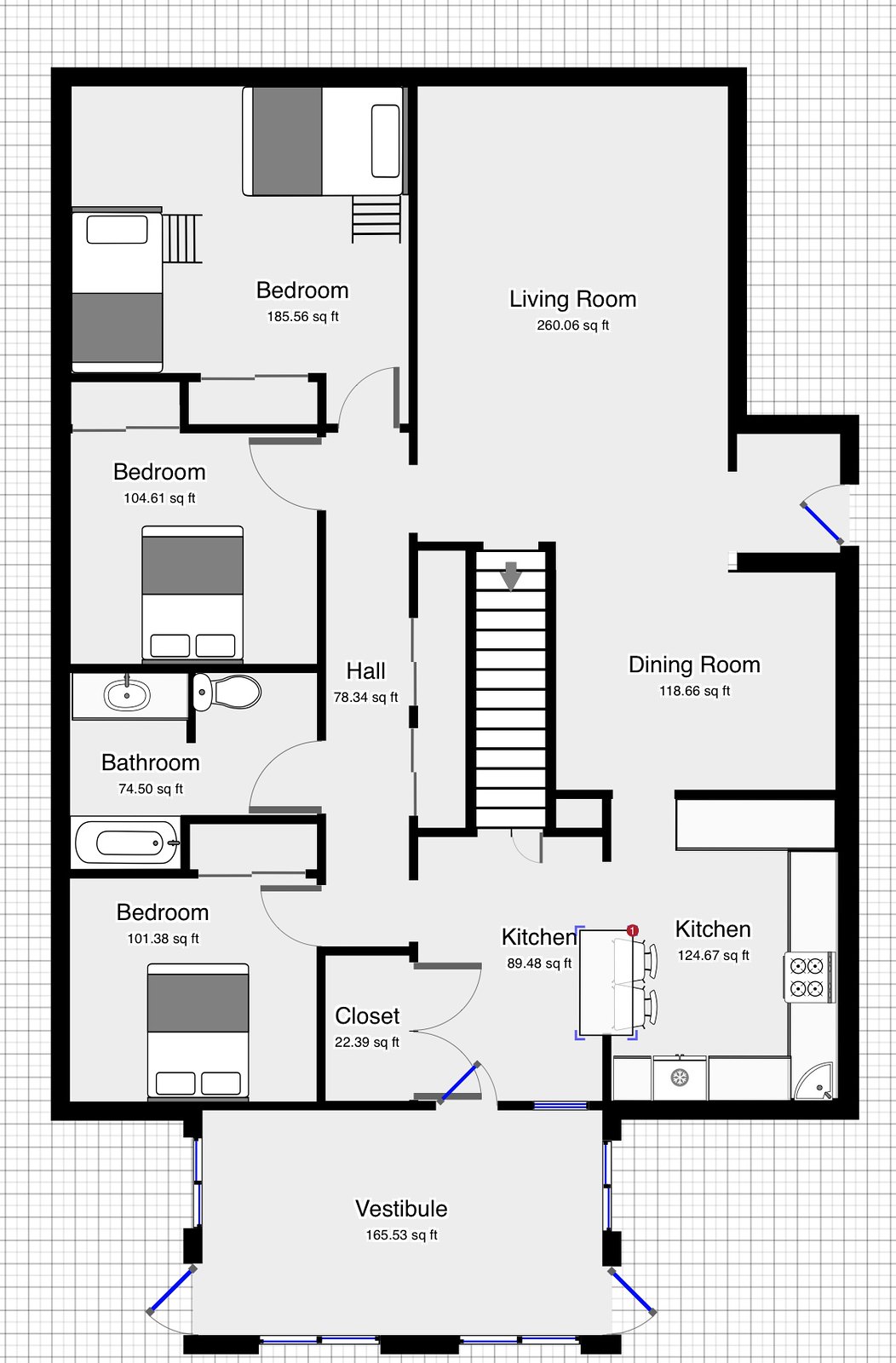This schematic illustrates a detailed floor plan of a housing unit, rendered on crosshatched drafting paper featuring varying shades of gray checks—darker gray, gray, and very light gray. The exterior walls are denoted by thick black lines, while blue lines indicate the presence of four exterior doors. Interior walls are marked with thinner black lines, and interior doors are shown as gray lines.

The layout includes a staircase with an arrow, suggesting a change in elevation, possibly leading to a basement. In the lower right-hand corner, the kitchen area features an island accompanied by two benches. Adjacent to the kitchen, there is a large entry closet and a vestibule, which functions as a sunroom.

In the left-hand corner sits a bedroom, beside which lies a shared bathroom that connects to another bedroom, emphasizing a three-bedroom layout. The living space comprises a living room and a dining room, providing communal areas for social interaction. 

This cozy, three-bedroom, one-bathroom home does not include a master suite but offers a practical and inviting living environment with a blend of functional and social spaces.